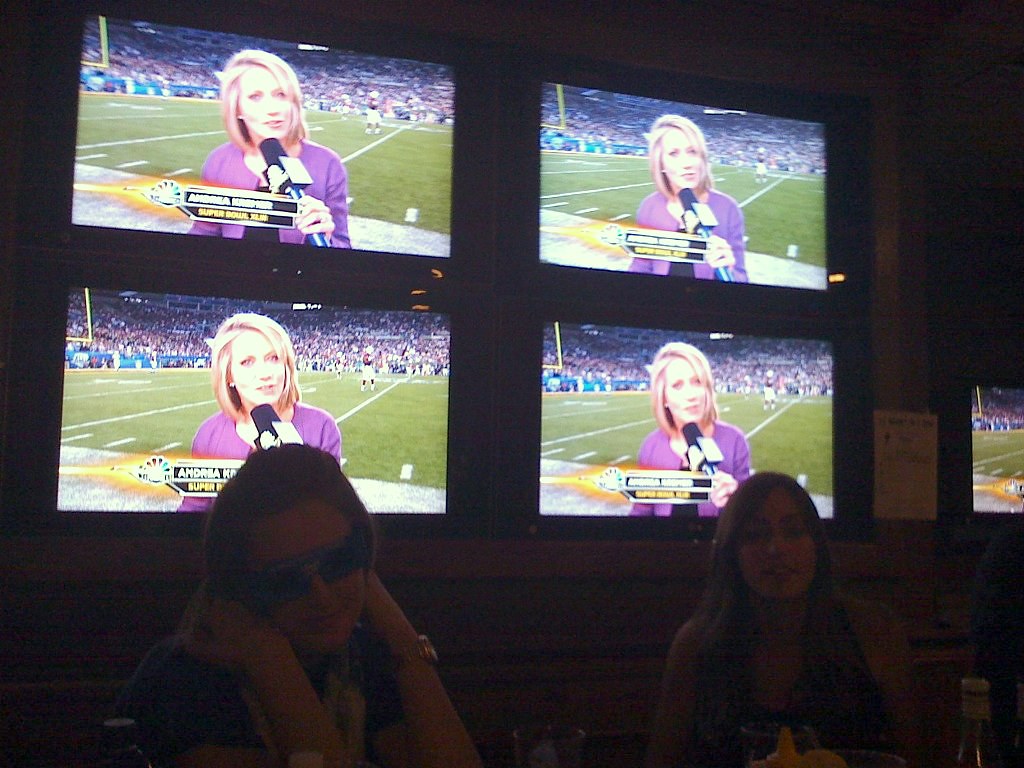In a dimly-lit sports bar likely dating from the early 2010s, two women sit at a table enjoying their evening. One woman, situated on the left, has long dark hair and wears a watch and sunglasses indoors. She holds her shoulder while glancing at the camera. The other woman, slightly older with short hair, also gazes into the camera with her lips slightly parted. Scattered remnants, such as a beer bottle on the table, suggest they may have just started their meal or drinks.

Behind them, four bright HDTVs dominate the scene, contrasting with the otherwise dark ambiance. The TVs display a sports broadcast, specifically an MSNBC Super Bowl coverage featuring a reporter named Andrea, dressed in a purple shirt and black blouse. The football field, crowded with spectators and players, stretches out behind her on the screen, adding to the lively atmosphere of the bar.